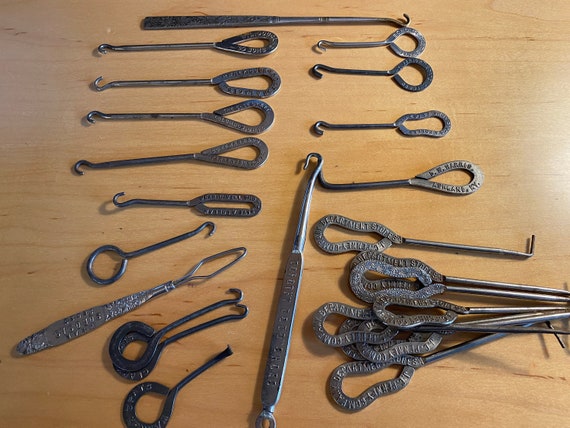This photo showcases a collection of assorted antique tools meticulously laid out on a blonde wooden table. Each tool is made from what appears to be hammered iron or steel and is characterized by a loop handle, either circular or oblong, followed by a long rod ending in various hook shapes or right-angle bends. The implements vary in length and design, with some terminating in a bulbous shape, while others end in sharp hooks. Though the specific use of these tools is unclear, they may be old-school dental instruments, crochet hooks, or early dermatological devices. Many of the tools carry stamped text on their handles, resembling a manufacturer's mark, but the letters are difficult to discern. The ornate craftsmanship and evocative design, reminiscent of a coiled snake, suggest these are not merely functional but also visually distinctive antique tools.